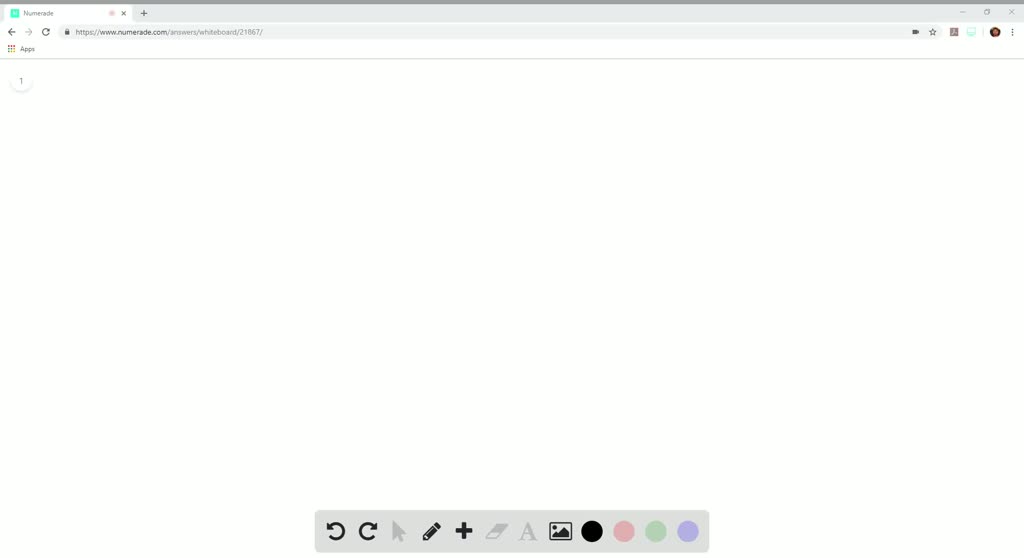A detailed snapshot of an internet browsing web page, depicting an unidentified browser window which could either be Chrome, Internet Explorer, or Safari. At the top, there is a light gray thin bar displaying only one tab, though its text is unreadable. Below the gray bar is an address bar with an active URL. The main section of the screen is completely blank, showing a white background with no content. At the bottom of the page, there is a gray toolbar suggestive of an illustration application, featuring several icons: undo, redo, a crayon symbol for drawing, a plus symbol, an image import icon, and four colored dots in black, pink, green, and purple.